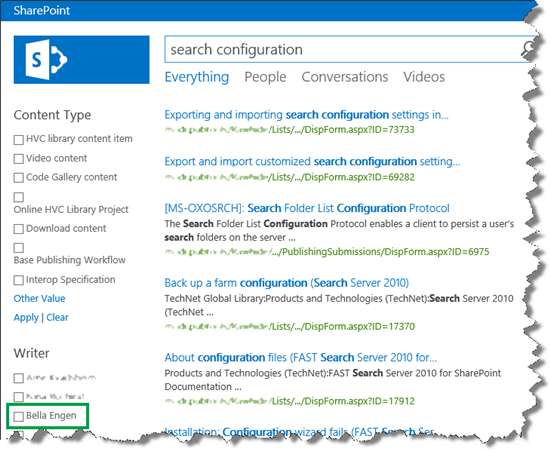This screenshot displays a window with an irregular, jagged, ripped paper effect along the right-hand side and bottom, suggesting it was crudely captured, possibly using a snipping tool. At the very top of the image, a thin royal blue bar contains the word "SharePoint" on the left. Directly below this bar is a small blue rectangle with the SharePoint logo.

In the main section of the window, there is a vertical column on the left labeled "Content Type." This column lists several items that can be checked, though none are currently selected. The items include:
- HVC Library Content
- Item Video Content
- Code Gallery Content
- Online HVC Library Project
- Download Content Base
- Publishing Workflow
- Interop Specification
- Other Value
- Apply
- Clear

Adjacent to this column is another column labeled "Writer," where two names are blurred out, but the third name visible is "Bella Engen," highlighted in a green box.

At the top right of the window, a search bar is labeled "Search Configuration," with search options for "Everything," "People," "Conversations," and "Videos," all highlighted in blue. Below this, several items related to search settings are listed, including:
- Exporting and importing a search configuration
- Export and Import Customize Search Configuration Setting
- MS-I-OXOSRCH Search Folderless Configuration Protocol